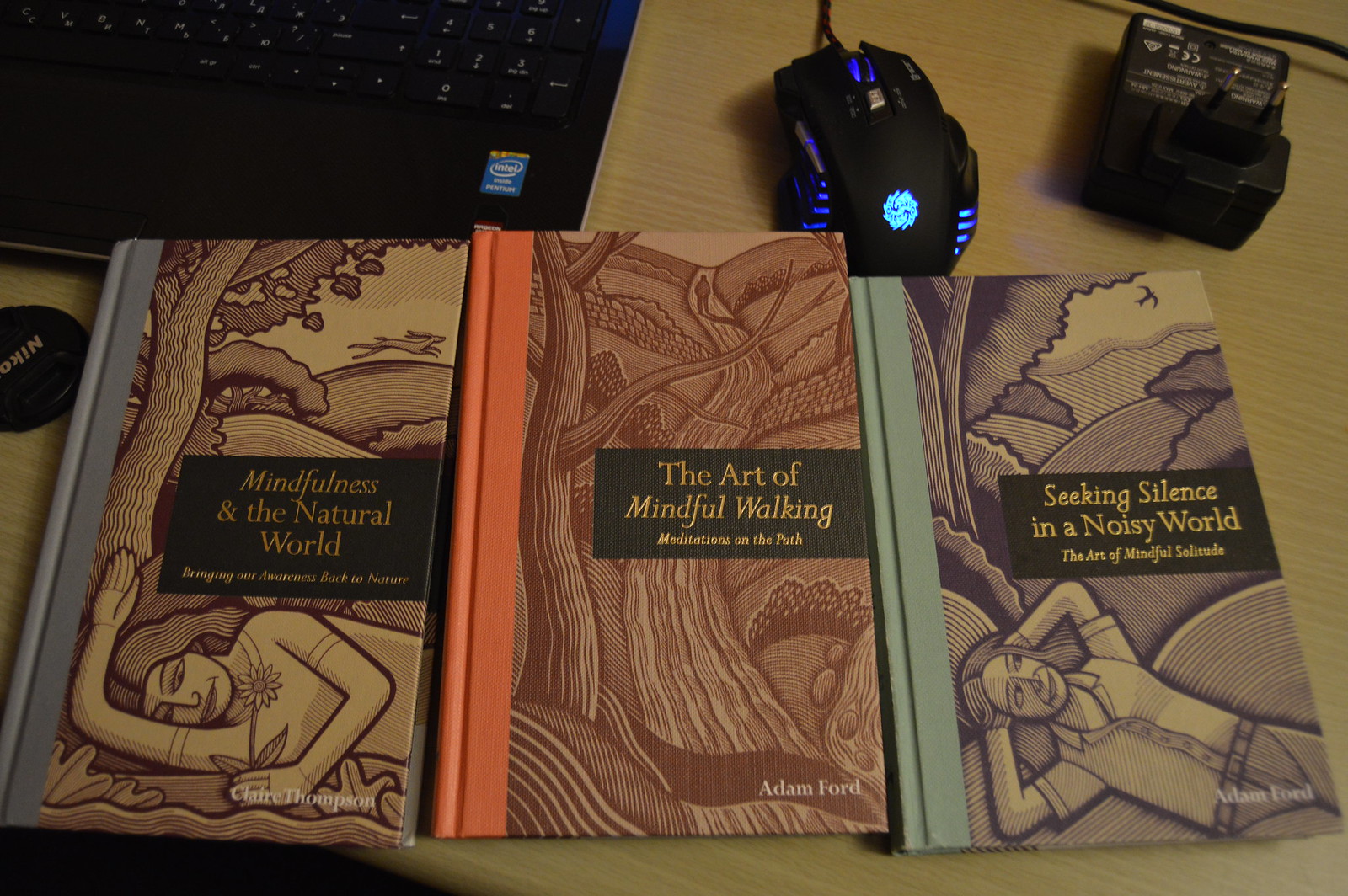The photo captures a top-down view of a golden brown wooden desk adorned with various items. In the upper left corner sits a black computer keyboard, accompanied by a sleek black mouse illuminated with blue lights. Beside the mouse lies a Nikon lens cap. Below the keyboard is a neatly arranged row of three hardcover books, each appearing to be part of a series focused on mindfulness.

The book on the left is "Mindfulness in the Natural World" by Claire Thompson, featuring someone laying on the ground on its cover. The middle book, "The Art of Mindful Walking: Meditation on the Path" by Adam Ford, displays an orange section. The third book, "Seeking Silence in a Noisy World: The Art of Mindful Solitude," also by Adam Ford, shows another image of someone laying on the ground. The spines of the books showcase different colors: blue, orange, and turquoise, from left to right.

In addition to these main elements, there is an unidentifiable object located near the mouse, and something that plugs into the wall is also visible among the items on the desk. The overall scene is one of a meticulously organized space centered around themes of mindfulness and digital work.